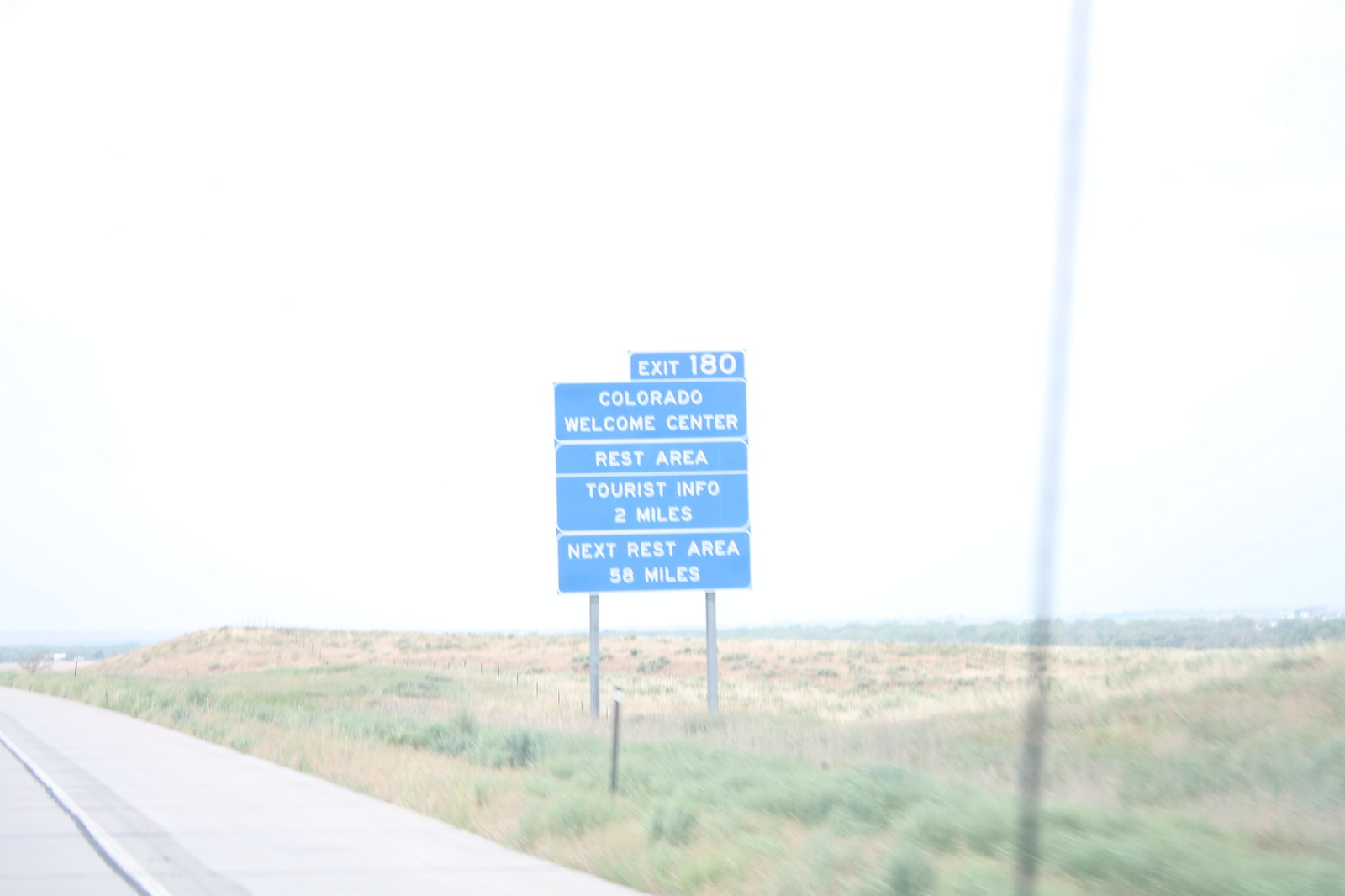In the image, a bright and clear sky stretches across the horizon, illuminating a landscape predominantly covered in dry grass. On the left side of the scene, a paved road extends into the distance. A striking blue sign, supported by two metal posts, captures attention in the foreground. The sign features white text that reads, "Exit 180, Colorado Welcome Center," followed by "Rest Area, Tourist Information 2 miles," and "Next Rest Area, 56 miles." In the far distance, the horizon is a vast expanse of dry grasslands interspersed with patches of darker green vegetation.